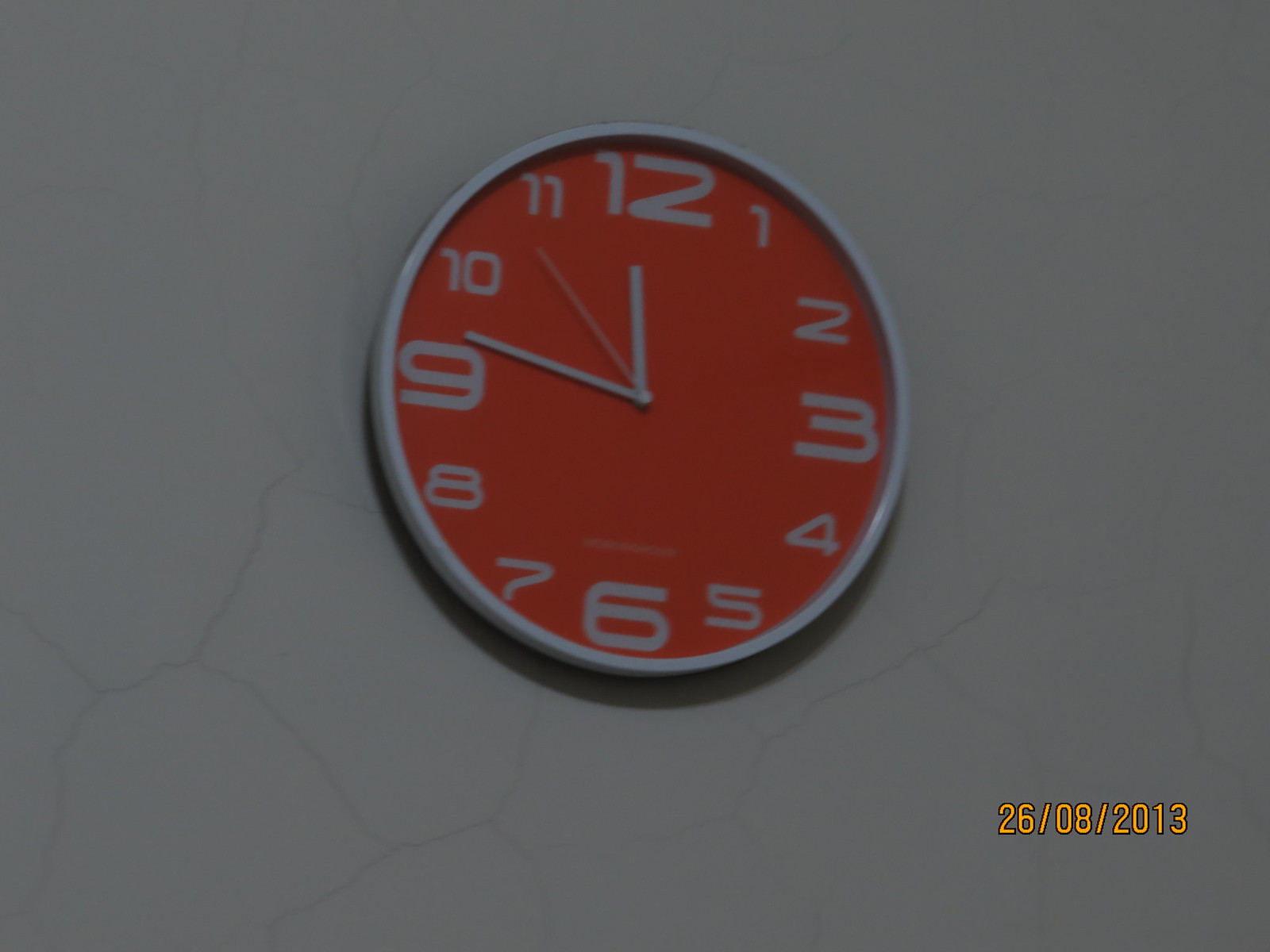This detailed image captures a distinctive red-orange clock mounted on a dark gray, heavily cracked wall, likely marred by an event like an earthquake. The clock hangs about an inch from the top and is centered on the wall. It casts a subtle shadow beneath it. The clock features gray numbers from 1 to 12, with the 12, 3, 6, and 9 being larger than the others. Additionally, the clock has two thick gray hands indicating the time is 11:46, with the longer hand just above the 9 and the shorter hand at the 12. A third, thinner hand lies between the 10 and 11 positions. Notably, in the bottom right corner of the wall, around two inches up, the date "26-08-2013" is clearly displayed in yellow.